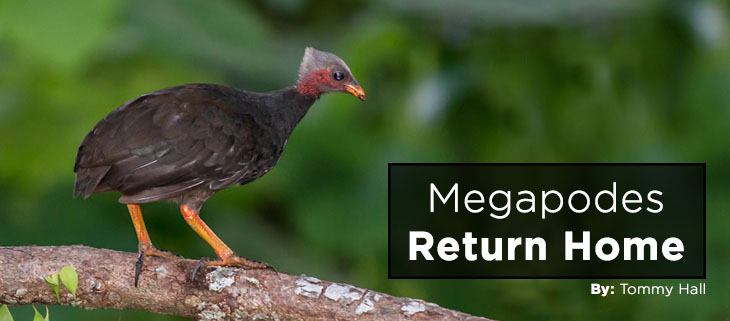In this image, we see a photograph that appears to be the cover of a book. The scene is set outdoors with a blurred green and gray background, suggesting trees or bushes. Dominating the foreground is a detailed side view of a bird standing on a tree branch that stretches from the right to the left. The bird, which is relatively small, has a dark brown body and orange-yellow legs with three toes. Its head is light gray with a noticeable red patch on the cheek that extends slightly down the neck, and an orange beak. The bird faces right, drawing attention to the text on the right-hand side of the image. This text is set in a brown rectangle with white lettering that reads "Megapodes Return Home." Below this title, also in white letters, is the author's name, "By Tommy Hall."